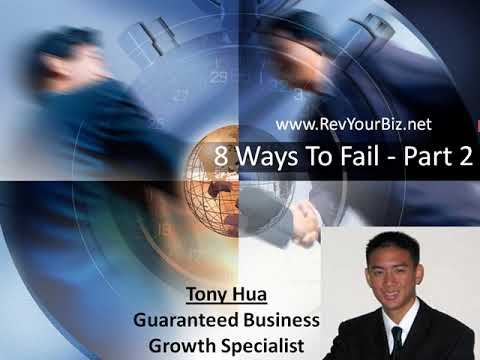The image is divided into four sections, featuring a central theme related to business. In the bottom-right quadrant, there is a clear, professional portrait of a young Asian man named Tony Hua. He has short, clean-cut black hair and is dressed in a black suit, white dress shirt, and black tie, all set against a white background. The text beside him identifies him as a "Guaranteed Business Growth Specialist."

The rest of the image comprises three additional sections. The two upper sections depict a blurry and abstract representation of two men shaking hands amidst a swirling bluish background, suggestive of a business agreement or partnership, with lines dividing the segments. In the center segment, there is a wireframe globe rendered in brown, giving a sense of global reach or connectivity. 

In the upper-right corner of the image, there is text that reads "www.revyourbiz.net, Eight Ways to Fail - Part Two," indicating that this is part of a business educational series or presentation, likely focusing on growth strategies and pitfalls.

The overall color palette of the image includes white, dark blue, bronze, brown, black, and some green hues, contributing to its modern and professional aesthetic. This digitally created piece emphasizes business growth, global connections, and professional advice, with Tony Hua as the focal point.